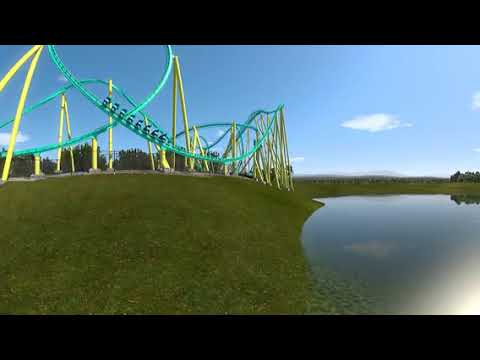In this detailed depiction, the image portrays a vibrant daytime scene at an amusement park, focusing on a striking roller coaster set against a picturesque backdrop. The roller coaster features a turquoise track intricately supported by thin yellow beams and appears to have thrilling loops and tall drops. This exciting structure dominates the left side of the frame, stretching over a vast, well-maintained grassy field. There is an element of uncertainty about the presence of people due to the image's somewhat clean and polished appearance, which lends a 3D-rendering feel, though it is likely a realistic photograph.

To the right of the roller coaster, there lies an eerily still body of water, reflecting the sunlight and adding a serene contrast to the surrounding activity. Beyond the tranquil lake, small mountains rise in the distance, accompanied by scattered trees both near the roller coaster and on the horizon. The sky is a clear blue with a few scattered clouds, enhancing the overall crispness of the scene. This photograph beautifully captures the juxtaposition of man-made excitement with the calm of nature, under a bright, clear sky.